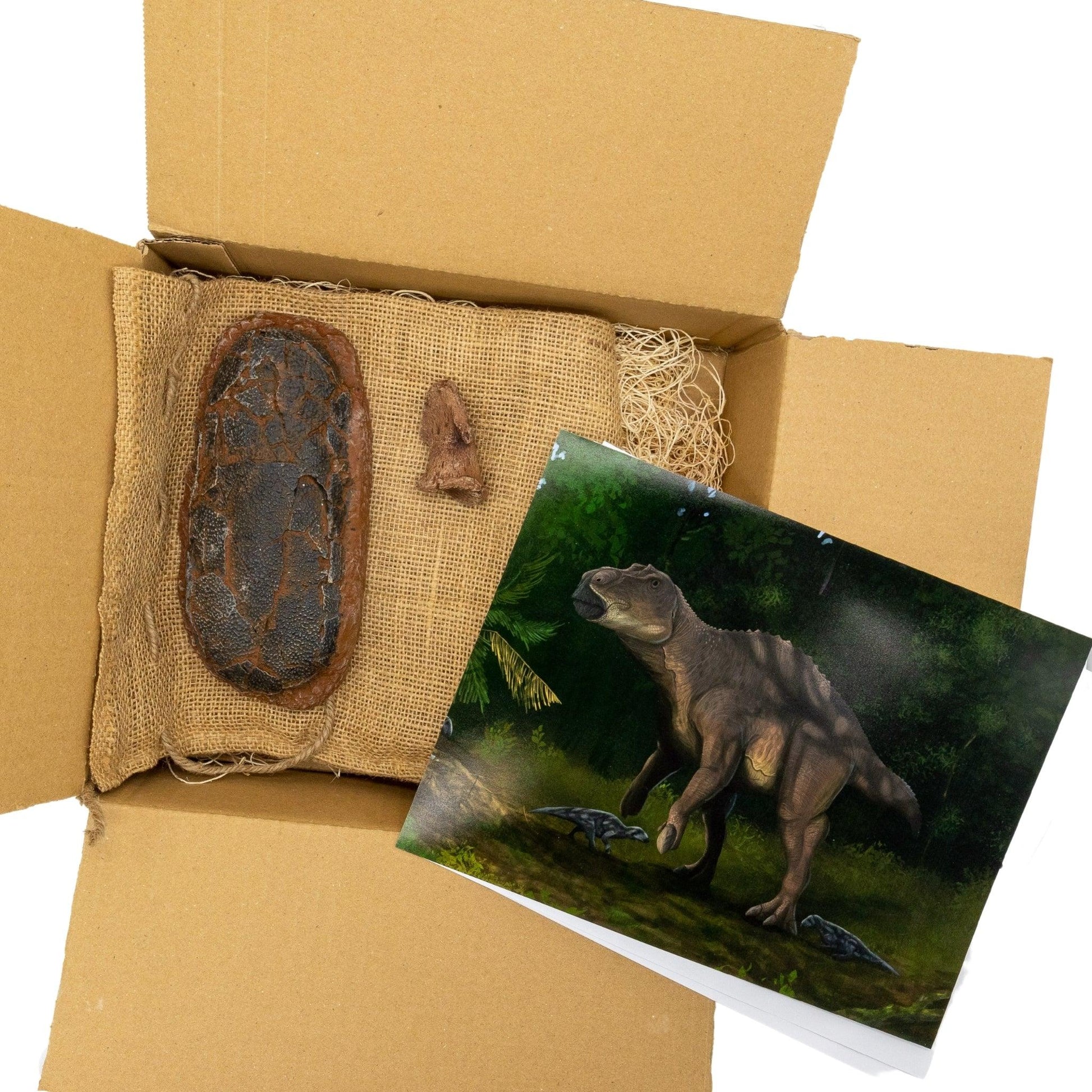The image depicts an overhead view into an open cardboard box set against a white background. All four flaps of the box are spread open, revealing its contents. Resting on the lower right flaps is a photograph or painting of a dinosaur, characterized by its large, robust legs, comparatively shorter arms, and a relatively short tail. This dinosaur is depicted alongside two baby dinosaurs in a forest setting. Beneath the photograph, a few loose, indeterminate papers can be seen.

Inside the box lies a brown, potato sack-like fabric at the bottom, partially covering what appears to be straw. Positioned atop this fabric are two dark brown rocks, varying in size, which could be archaeological artifacts related to the dinosaur in the photograph. The scene suggests a connection between the rocks and a paleontological theme, possibly hinting at them being fossils or remnants linked to the era of the depicted dinosaurs.